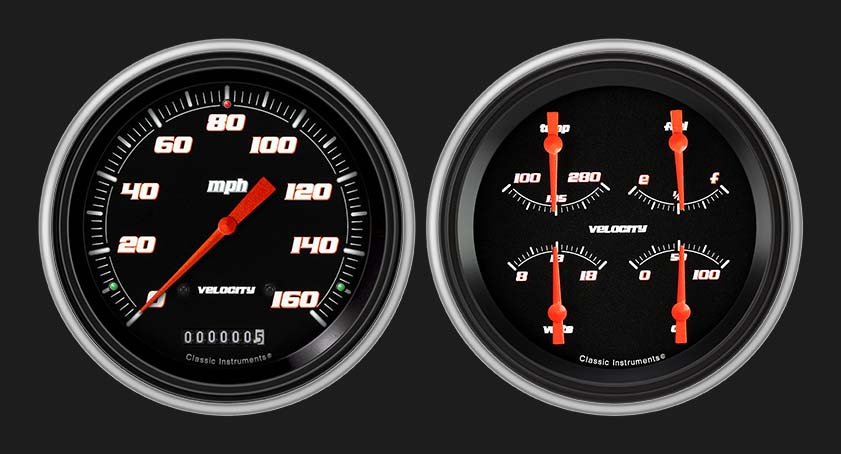The image depicts an intricately detailed illustration of a car's instrument panel. Set against a black backdrop, the panel features two circular gauges encased in grey borders. The gauge on the left is a speedometer with a red arrow pointing to zero miles per hour. White numerical markings surround the speedometer, indicating speeds from 0 to 160 miles per hour in increments of 20. Below the speedometer, the odometer displays "000,000.5" miles, and "Classic Instruments" is inscribed at the bottom. The instrument on the right is a multi-functional gauge divided into four sections, each with its own orange arrow pointing to the center of the respective meter. These sections include a temperature gauge ranging from 100 to 280, a fuel gauge marked from E (Empty) to F (Full), a voltmeter ranging from 8 to 18 volts, and another gauge numbered from 0 to 100. This sophisticated graphic design perfectly mimics the layout of a real car dashboard, offering a comprehensive view of essential vehicular metrics.